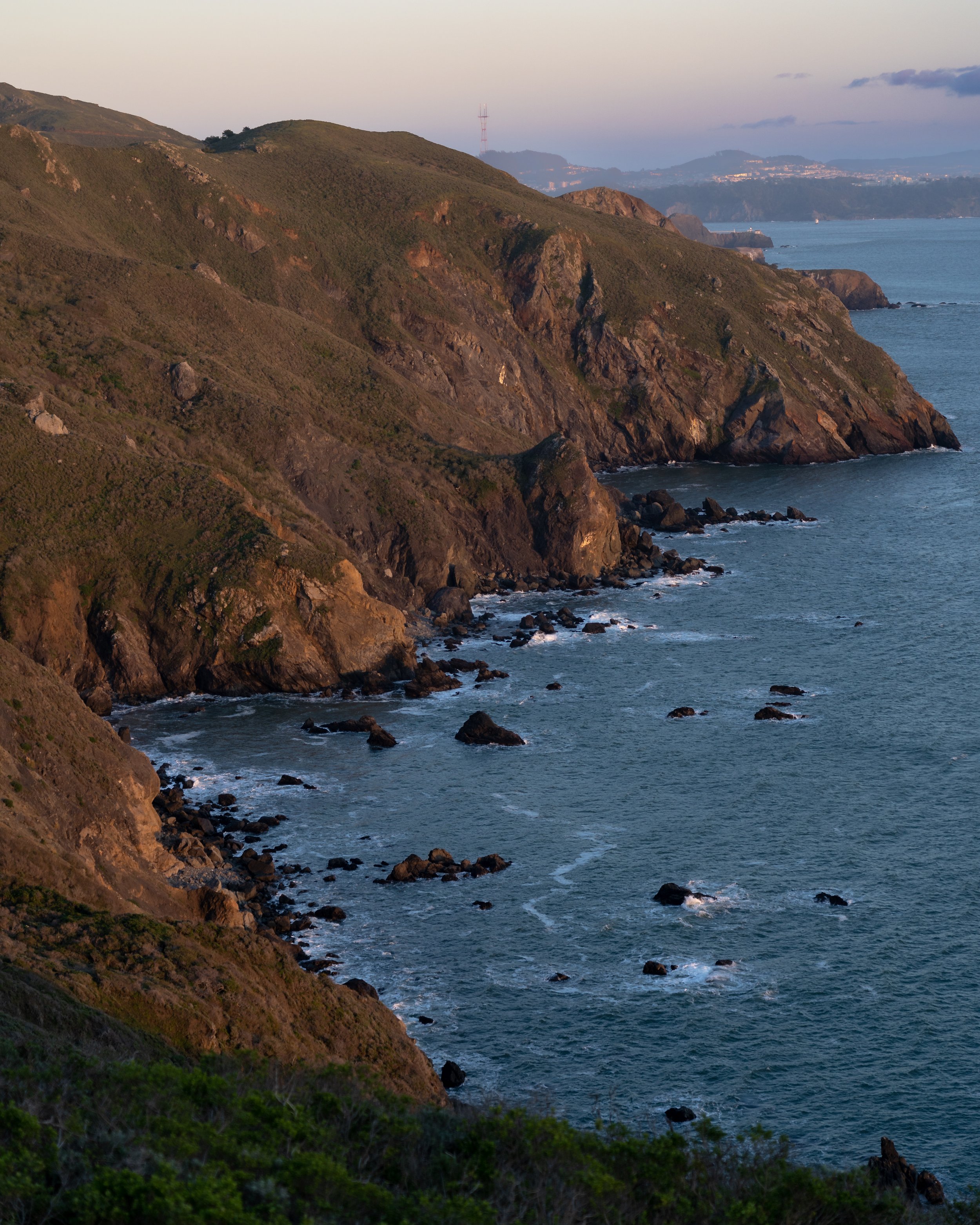This photograph captures a rugged shoreline, where the land transitions sharply into the water with jagged, rocky edges rather than a sandy beach. The scene is viewed from a grassy hill that slopes gently towards the water, contrasting with the predominantly brown, sparsely vegetated hills around it. The water, relatively calm with a few waves, shows white splashes at its rocky interface. Dotted throughout the water, numerous rocks punctuate the scene, hinting at the rough terrain beneath. In the far distance, across the body of water, another landmass punctuates the horizon, with a hint of greenery and ambiguous white structures that could signify a distant, hazy city. A prominent tower-like structure stands on this distant landmass, slightly to the top middle of the image. The backdrop boasts more mountainous terrain with some green brush in the foreground. The sky is a blend of light pink and blue hues, indicative of either sunrise or sunset, scattered with clouds. The overall palette of the image is rich in earth tones—browns, blues, greens, and grays—complemented by the soft, pastel sky. There are no human figures present, and the cliffs drop steeply into the water, with no apparent access route, underscoring the rugged and untouched nature of the landscape.